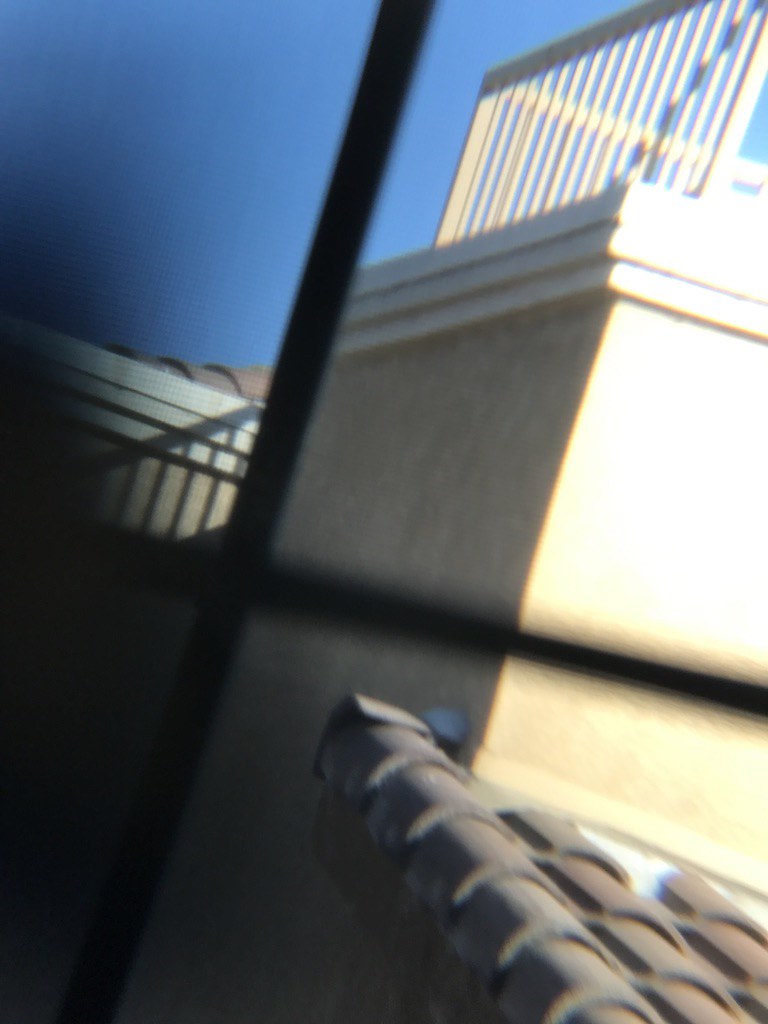This photograph captures an exterior view, likely taken through a window. The lower right-hand corner features a roof covered with ceramic or pottery tiles, arranged in an overlapping fashion. These tiles are cylindrical in shape and have a rich, brick-red color. Adjoining the roof is a tan-colored wall that meets at a visible corner. Atop this wall is decorative molding, and above that, there is a screened area, possibly part of a porch or balcony. Dominating the left-center of the image is a prominent window frame, which creates a large 'X' shape across the scene. The sky is a brilliant shade of blue, providing a vivid backdrop. However, a dark spot on the left side of the photograph obscures some details in that area.